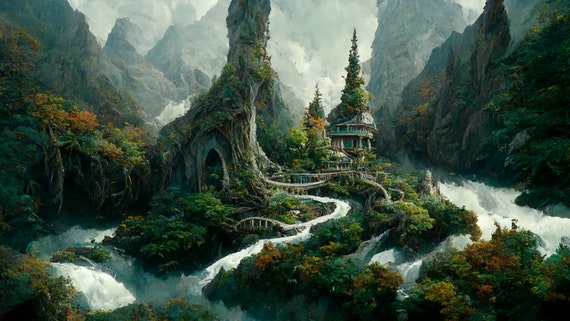In this conceptual fantasy image, a lush, intricate city nestles within a verdant forest valley flanked by mountains on either side. The scene is dominated by an array of green, white, and a hint of orange and brown, creating a vibrant yet chaotic palette. The city's most striking feature is a tiered, domed structure on the right, seemingly interwoven with nature as a tree emerges from its roof. Pathways wind through the area, alongside a dynamic river that courses through the landscape with rapid intensity. Central to the image is a towering tree with a gothic arch carved into its trunk, suggesting a dwelling within. Bridges crisscross the scene, connecting various buildings that meld seamlessly with their surroundings, covered in lush vegetation, creating the appearance of an organic, living architecture. The gray sky above, laced with messy, vertical lines, adds a contrasting background to the vivid greens and fluffy, cloud-like clusters that punctuate the image, intensifying the mystical, otherworldly atmosphere of this imagined haven.